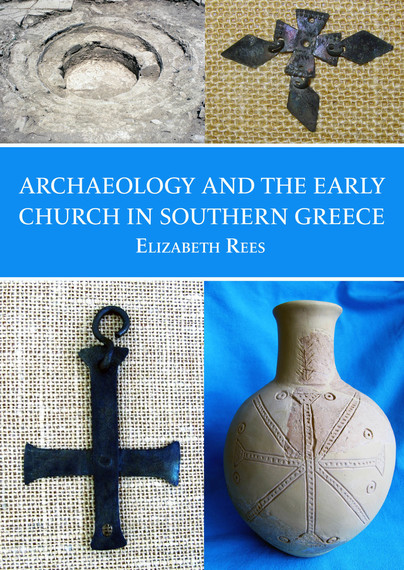The image depicts the cover of a book titled "Archaeology and the Early Church in Southern Greece" by Elizabeth Rees, prominently displayed in white text over a blue banner placed centrally on the cover. The cover is divided into four quadrants, each containing a photograph. The top left photo shows the circular, layered ruins of what appears to be an ancient amphitheater or stone pit. To its right, in the top right quadrant, is an artifact resembling a metallic cross or medallion with complex geometrical designs, set against a beige background. The bottom left quadrant features an inverted black cross with a hook extending from the top, against a canvas-like backdrop. Finally, the bottom right quadrant displays a beige amphora or clay vase, intricately decorated with etched patterns, and set on a blue fabric background, matching the blue banner of the title. The overall layout and illustrative nature of the cover suggest it might be an academic book, possibly a visually rich coffee-table book.